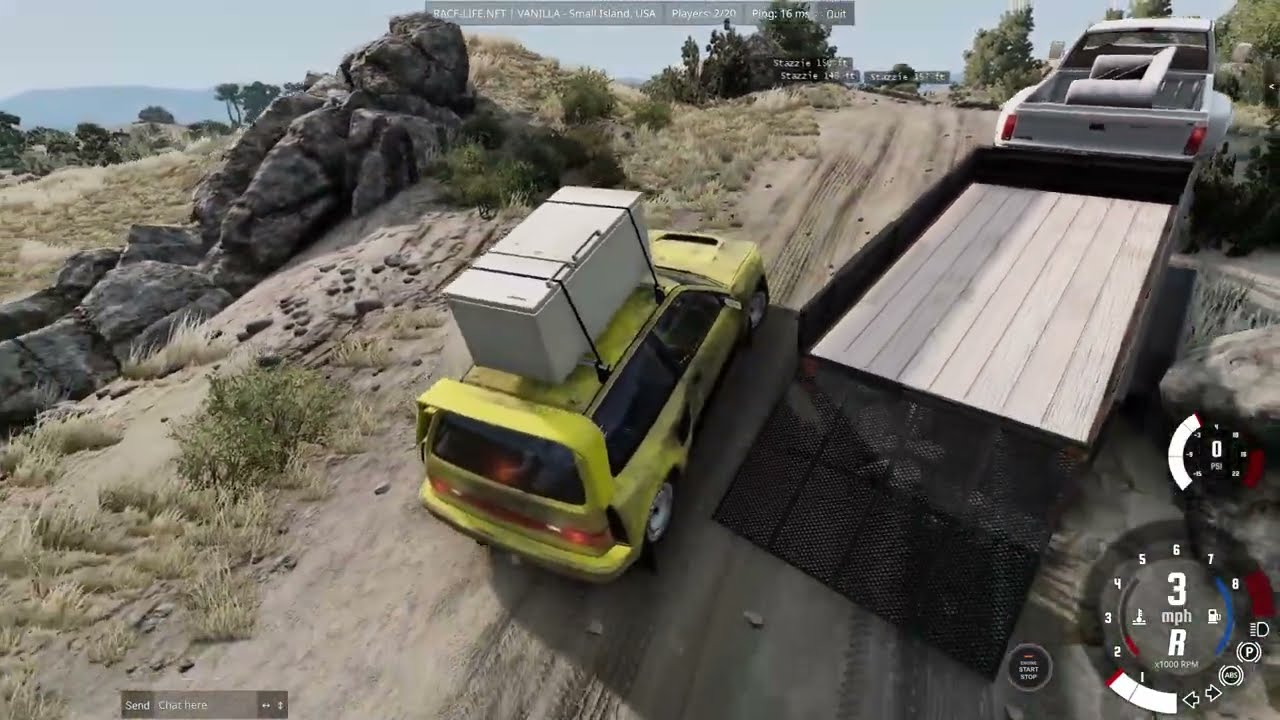This detailed screenshot from a driving video game captures a scene on a steep, dirt-covered hill with rocky terrain flanking both sides of the pathway. The right side of the road features a white pickup truck carrying a living room-style armchair in its bed and pulling a flatbed trailer with its ramp gate lowered, exposing the wooden flooring. Nearby, a beat-up yellow low-rise hatchback, presumably an SUV, is shown overtaking the truck while hauling a refrigerator strapped to its roof, along with a large yellow fan at the back. The vehicle appears worn and covered in dirt. The game's interface is visible on the screen, with a speedometer and tachometer gauge located in the bottom right corner alongside a start-stop button, and car instrumentation indicators like parking and headlights. The top of the screen displays text reading "racelife.net Vanilla small island USA players 2 out of 20 ping 16 ms" followed by a quit option. The hilly environment is accented with patches of greenery and sand, suggesting a semi-desert setting with mountainous backgrounds.